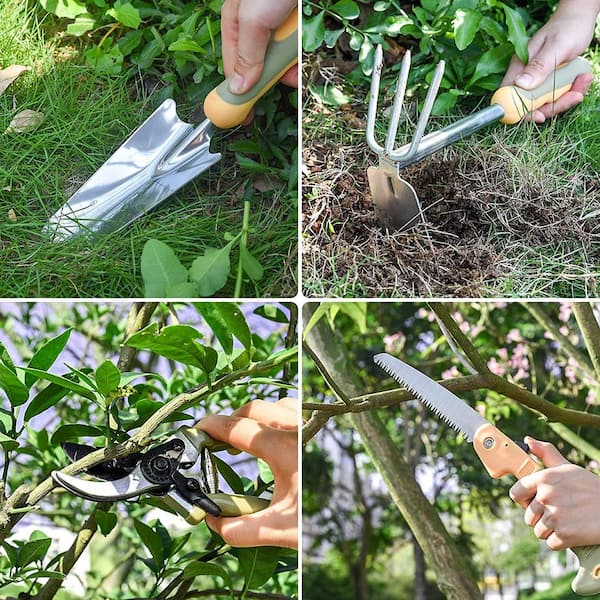This is a series of four uniformly sized photographs arranged in a square, each depicting a different gardening tool held by a human hand in the act of gardening. 

1. The upper left quadrant features a shiny chrome-colored trowel with an orange handle, being pressed into vibrant green grass.
2. The upper right quadrant showcases a dual-purpose hand tool with a flat trowel and three short rake-like claws, held against some withered, grayish-brown grass.
3. The lower left quadrant displays a pair of snipping tools, poised to cut through a small leafy branch, hinting at a spring or summer setting.
4. The lower right quadrant shows a small handsaw with an orange handle, positioned against a somewhat thicker branch, ready for cutting.

These images collectively emphasize various gardening activities, set against the green backdrop of a garden environment.